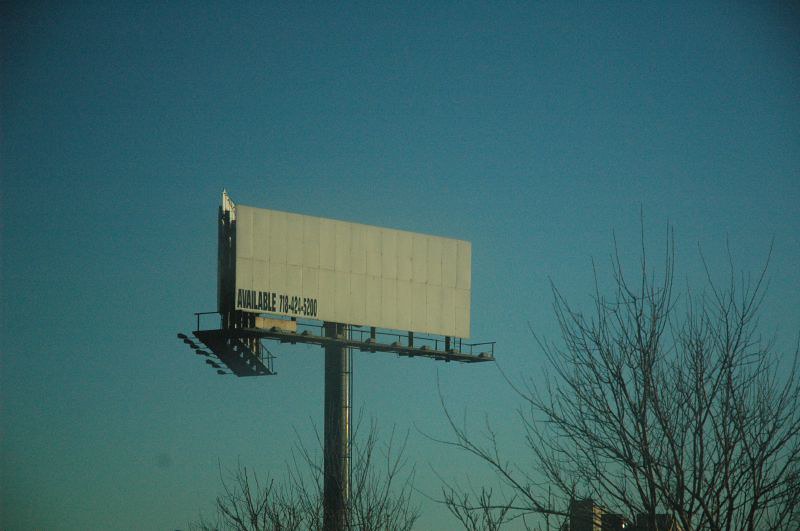The image features a blank white billboard mounted on a large metal post, photographed from a low angle looking upward. The billboard displays black text at the bottom left that reads "Available" followed by a phone number, 718-424-5200. This metal post has a ladder built into it and is designed with mounted lights to illuminate the billboard. In the background, a cloudless blue sky provides a backdrop, while the tops of barren trees, their branches devoid of leaves, suggest the scene is captured during winter. Towards the left side of the image, the side view of another billboard is partially visible. Near the lower part of the image, there are hints of additional structures and possibly a chimney, adding to the scene's complexity.